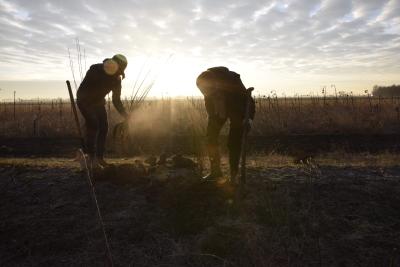In this outdoor scene, the sky is filled with light blue hues and scattered white clouds, with the sun peeking through and casting a clear, bright light over the landscape. The field below, mostly barren and brown with some patches of weeds, suggests a wintry or early spring setting. Two individuals, both silhouettes due to the brightness of the sun behind them, are at the center of the image, appearing to be engaged in some activity, possibly digging or picking at the ground with shovels or sticks. They are dressed in winter clothing, which is difficult to make out in detail. There is a mound of something ambiguous between them, possibly obscured by the poor image resolution, along with some indications of taller plants like hay or wheat in the background. The horizon features a distant line of trees, and the overall atmosphere evokes a sense of hard, earnest labor set against the serene backdrop of nature transitioning seasons.